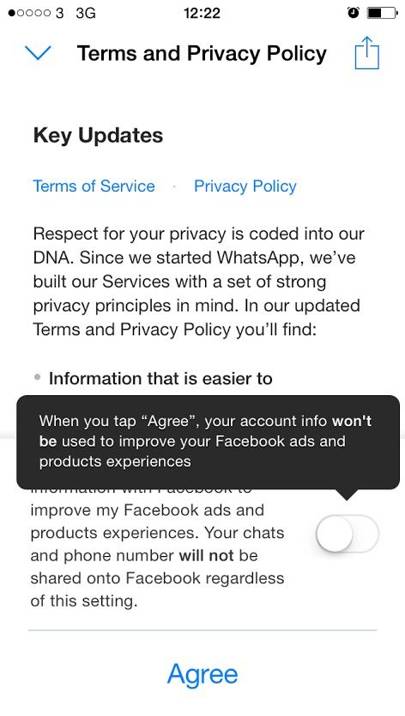The image appears to be a cropped mobile screenshot, leaving the operating system indeterminable. The top left corner shows signal strength bars represented as one black circle and four white circles, indicative of cellular connectivity rather than circles. The text "3" followed by "3G" suggests an older network standard, which may point to a dated screenshot or one from an area without advanced network technology. The time displayed is 12:22, although the distinction between AM or PM is not provided. An alarm is set, and the battery is approximately at 50% charge.

Within the screenshot, a downward blue arrow directs attention to the next section, where "Terms and Privacy Policy" is boldly presented in black. Adjacent to this, a share icon (a square with an arrow emerging from it) is visible. Below, the heading "Key Updates" is featured in black font, with interactive links for "Terms of Service" and "Privacy Policy" in blue.

The text below states: "Respect for your privacy is coded into our DNA. Since we started WhatsApp, we've built our services with a strong set of strong privacy principles in mind." In updating their Terms and Privacy Policy, WhatsApp aims to provide clearer information, though the exact details are obscured by a pop-up. This overlay explains that upon tapping 'Agree', account information won’t be used to enhance Facebook ads and products, and emphasizes that chats and phone numbers will not be shared with Facebook, independent of the setting.

A blue "Agree" button is positioned at the bottom of this informational layer, prompting users to consent to the updated terms in order to continue using the WhatsApp service.

In summary, the screenshot captures WhatsApp's notification about updated Terms and Privacy Policy, urging user agreement to maintain service usage while ensuring the privacy of chat and phone number information from Facebook integration.